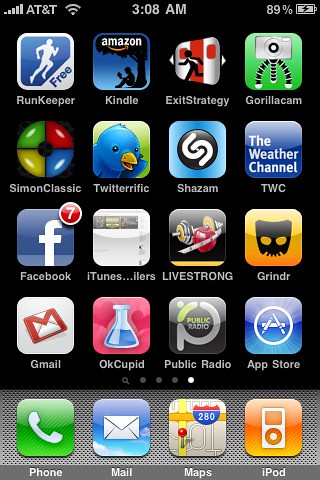This image is a detailed screenshot of an old iPhone home screen, highlighting the user interface and app arrangement typical of early iOS versions. At the top of the screen, the status bar shows the service provider as AT&T, with additional icons indicating a Wi-Fi connection and phone signal. The time displayed in the center of the status bar is 3:08 AM, and on the upper right corner, the battery life is shown at 89% with an indication that it is charging.

Following the status bar, the main interface reveals the apps organized in a precise 4x4 grid. In the first row of apps, starting from the upper left corner, are RunKeeper, Amazon Kindle, Exit Strategy, and GorillaCam. The second row contains Simon Classic, Twitterrific, Shazam, and The Weather Channel. The third row features Facebook, iTunes, Livestrong, and Grindr. Finally, the fourth row includes Gmail, OKCupid, Public Radio, and the Apple App Store. 

At the very bottom of the screen, the dock area houses the primary apps, arranged from left to right: Phone, Mail, Maps, and iPod. The overall design reflects the classic look and feel of one of the initial iPhone/iOS interfaces.